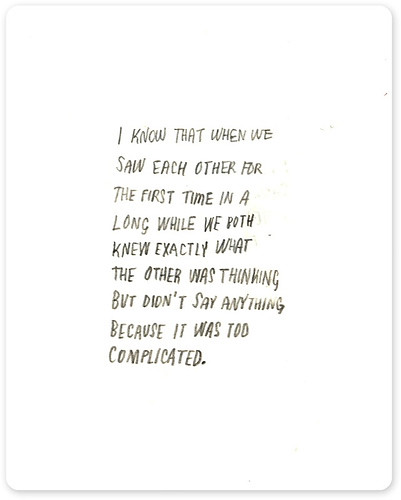The image features a vertical, white rectangle resembling a piece of paper, centered against a white background. It displays a quotation in a grayish-black, all-capitalized text that reads: "I know that when we saw each other for the first time in a long while, we both knew exactly what the other was thinking, but didn't say anything, because it was too complicated." The uneven and slightly smashed-in lettering gives the impression of being hand-printed, as it varies in darkness and lacks the uniformity of professional typesetting. The text occupies the center of the white background, with no additional drawings or elements present, emphasizing the raw, personal feel of the message.